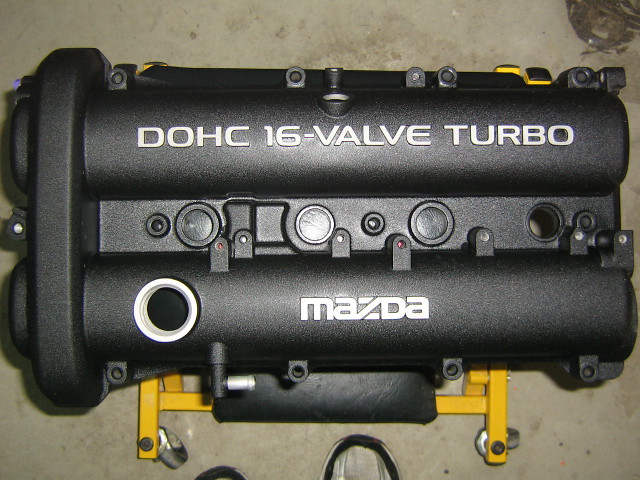The photograph presents a detailed overhead view of what appears to be an engine or an engine cover, labeled "DOHC 16 valve turbo" and "Mazda." The engine, colored in a dark charcoal gray or black chrome, is placed on a yellow-framed mechanics creeper, a low-profile cart typically used for lying down to slide under vehicles. The black padded seat of the creeper is partially visible under the engine. In the lower part of the image, we can see a pair of gym shoes, likely the photographer’s, positioned on a concrete garage floor. The photograph captures various valves, screws, and an oil fill tube on the left side of the engine cover, against the backdrop of a shop setting.